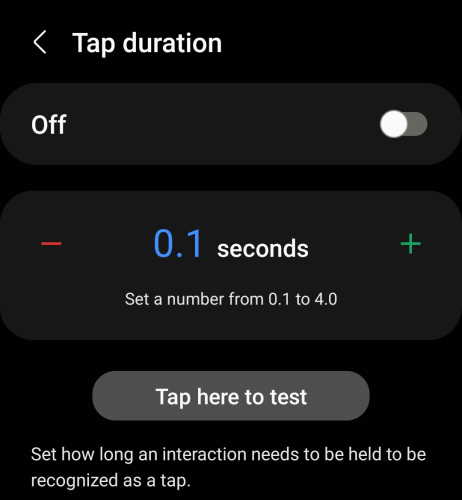The image showcases a screenshot of a black-and-white application interface with additional accents of green, blue, and red. At the top of the screenshot, a white left-pointing arrow is displayed next to the text "Tap Duration." Below this is an "Off" button, clearly indicated in white text on a grayish-black banner, with the toggle switch set to off and visible in white as well.

Further down, another banner in dark gray contains an adjustable setting for tap duration. A red minus sign, followed by the number "0.1" in blue seconds, and a green plus sign suggest a range that can be adjusted from 0.1 to 4.0 seconds. 

At the bottom of the interface, a light gray button labeled "Tap Here to Test" is present, along with additional instructional text: "Set how long the interaction needs to be held to be recognized as a tap."